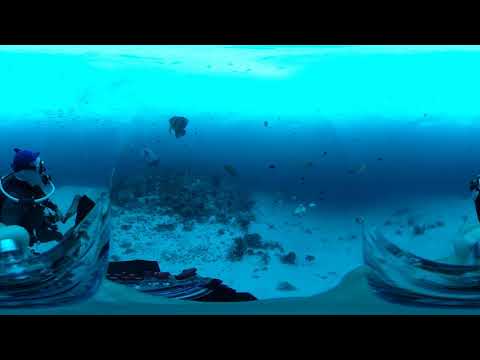The photograph captures an underwater scene, displaying a gradient of blue hues that transition from turquoise at the top to darker blue in the middle, before reaching a sandy ocean floor at the bottom. A scuba diver, equipped with a scuba tank, mask, goggles, and a snorkel, is situated on the far left side of the image, observing the aquatic life around them. The diver is attired in a black wetsuit and flippers. The scene includes various fish, some dark-colored, swimming across the image, and a large, prominent fish directly in front of the diver. Additionally, coral reefs and rocks, along with shells, can be spotted on the white sand at the bottom. The water is illuminated by sunlight penetrating the surface, creating layered blue tones. It appears the photograph might be a frame from a 360-degree video, given its possibly distorted and slightly blurry quality. Despite its low resolution, the detailed underwater composition vividly depicts the serene and lively oceanic environment.